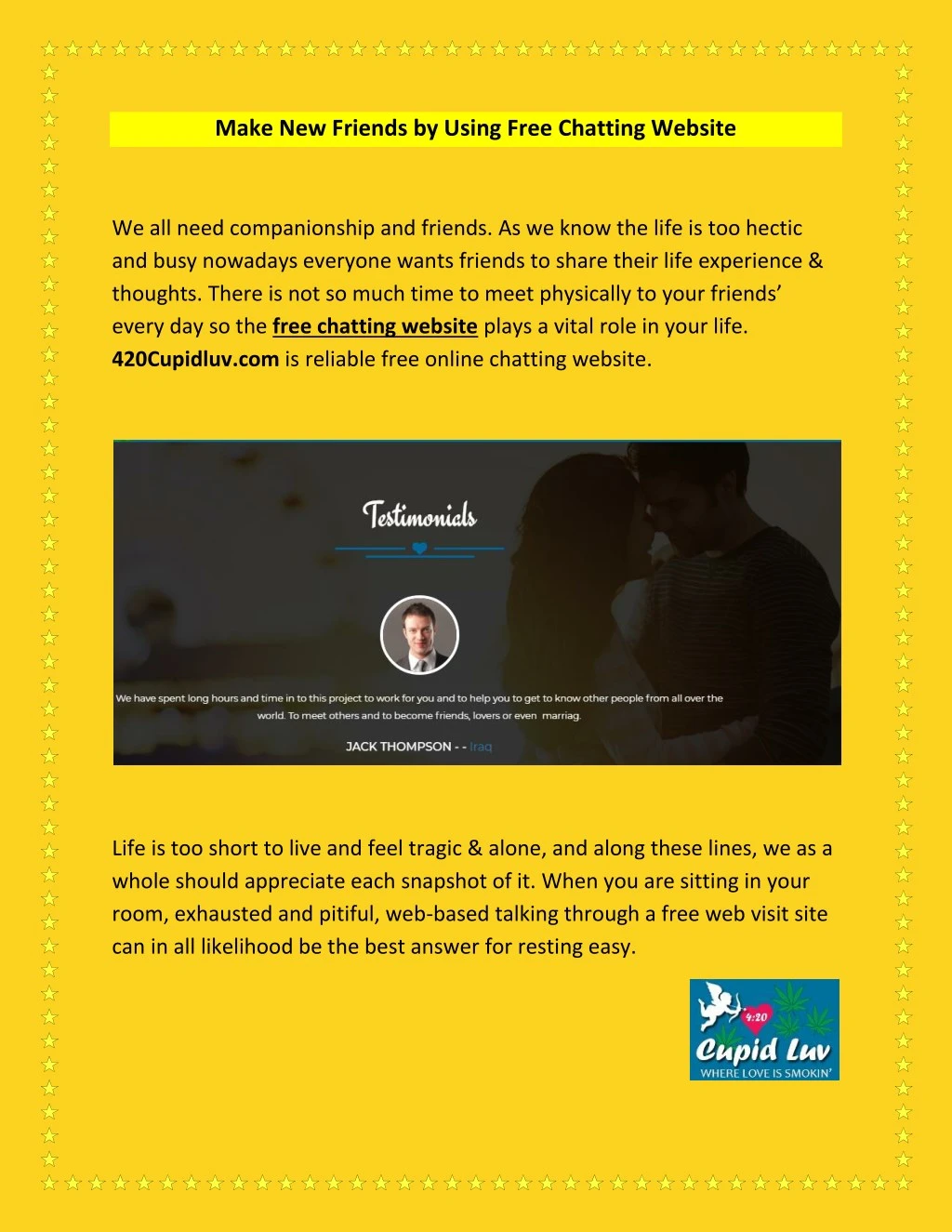Here's a detailed and cleaned-up caption for the described image:

---

A vibrant poster promotes a free chatting website, "port20cupidloveluv.com," set against a large yellowish-orange background adorned with a starry border. The message emphasizes the importance of companionship and friendship in today’s busy and hectic life, where finding time to meet friends in person daily is challenging. This reliable online platform offers the perfect solution for people seeking to share their experiences and thoughts. 

The center of the poster features a photo under the heading "Testimonials." The image displays a man in his 30s, dressed in a business suit, with a dim background picture of a smiling, cozy couple. The tagline, "Cupid Love, where love is smoking," adds a playful touch, further enhanced by an illustration of a cupid shooting a heart in the bottom right corner. Despite some grammatical and linguistic inaccuracies, the essence of the message—connecting people in need of companionship—remains clear.